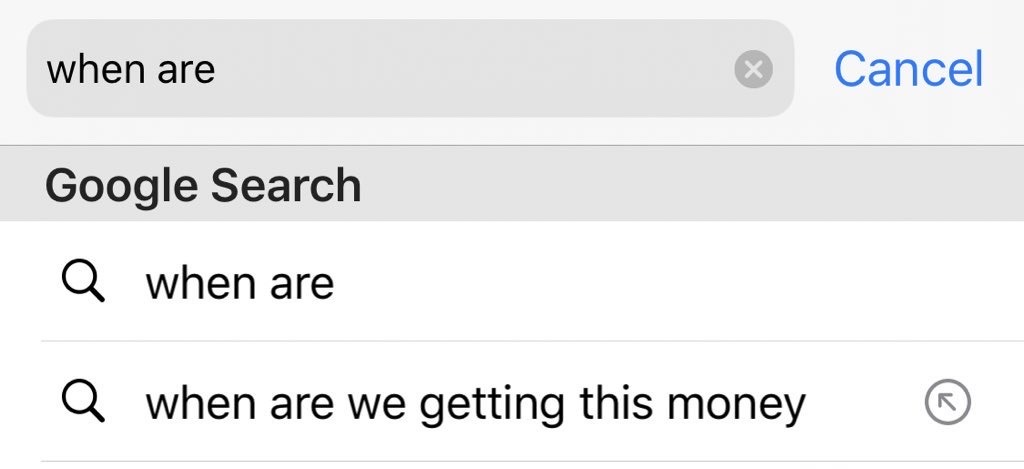The image depicts a web page with a predominantly white background. The interface features a gray search bar containing black text where the user has started typing the letter "R". Adjacent to the search bar is a blue cancel button with accompanying blue text. Above the search bar, a gray banner displays the text "Google Search" in black font alongside a black magnifying glass icon. Below, the search bar is divided by a gray separator line leading to another section containing a text input field. This field displays the query "when are we getting this money?" in black text next to a black magnifying glass icon. At the bottom of the image, another gray line delineates the lower portion of the page, featuring a circle with an arrow pointing diagonally to the side.